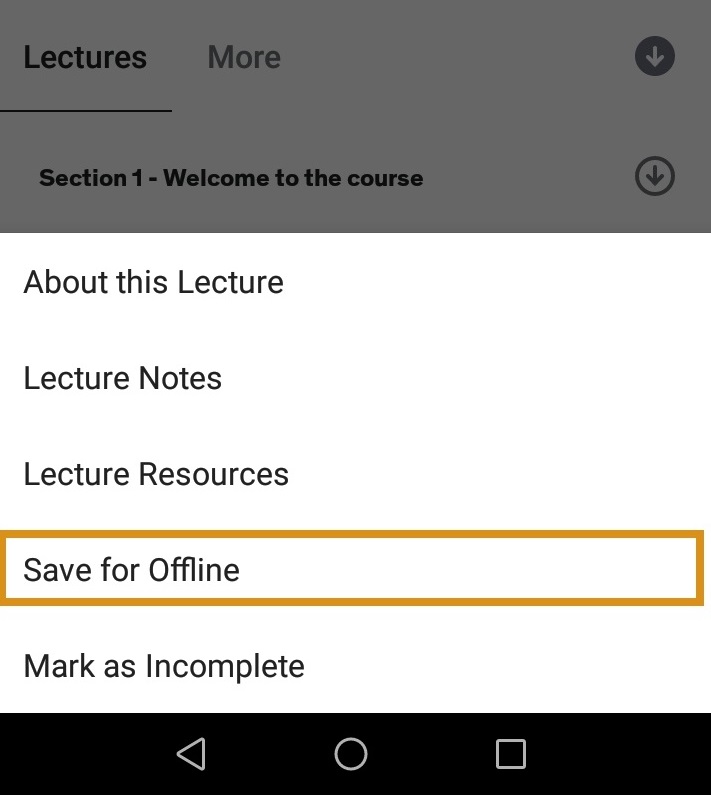The image is a rectangular screenshot of an educational app interface. In the top-left corner, the word "Lectures" is displayed prominently, and alongside it, in dark gray text, is the word "More". In the upper right corner, a circular dark gray icon featuring a white downward-facing arrow is visible. Just below, in bold black text, it reads "Section 1, Welcome to the Course". Adjacent to this text on the right side is another circular icon with a gray background, a dark gray outline, and a downward-facing dark gray arrow.

A menu is open beneath this heading. The menu, set against a white background with black text, lists several options: "About this Lecture", "Lecture Notes", "Lecture Resources", "Save for Offline", and "Mark as Incomplete". Notably, "Save for Offline" is highlighted in bright orange, drawing attention to this link.

Below the menu, a black bar spans the width of the image, seemingly forming the backdrop for navigational buttons. On the left side of this bar, there's a left-facing triangular light gray arrow, indicating a back button. Centrally placed is a circular button, likely for returning to the home screen. On the right side is a square button, designed to reveal all open windows on the user's phone.